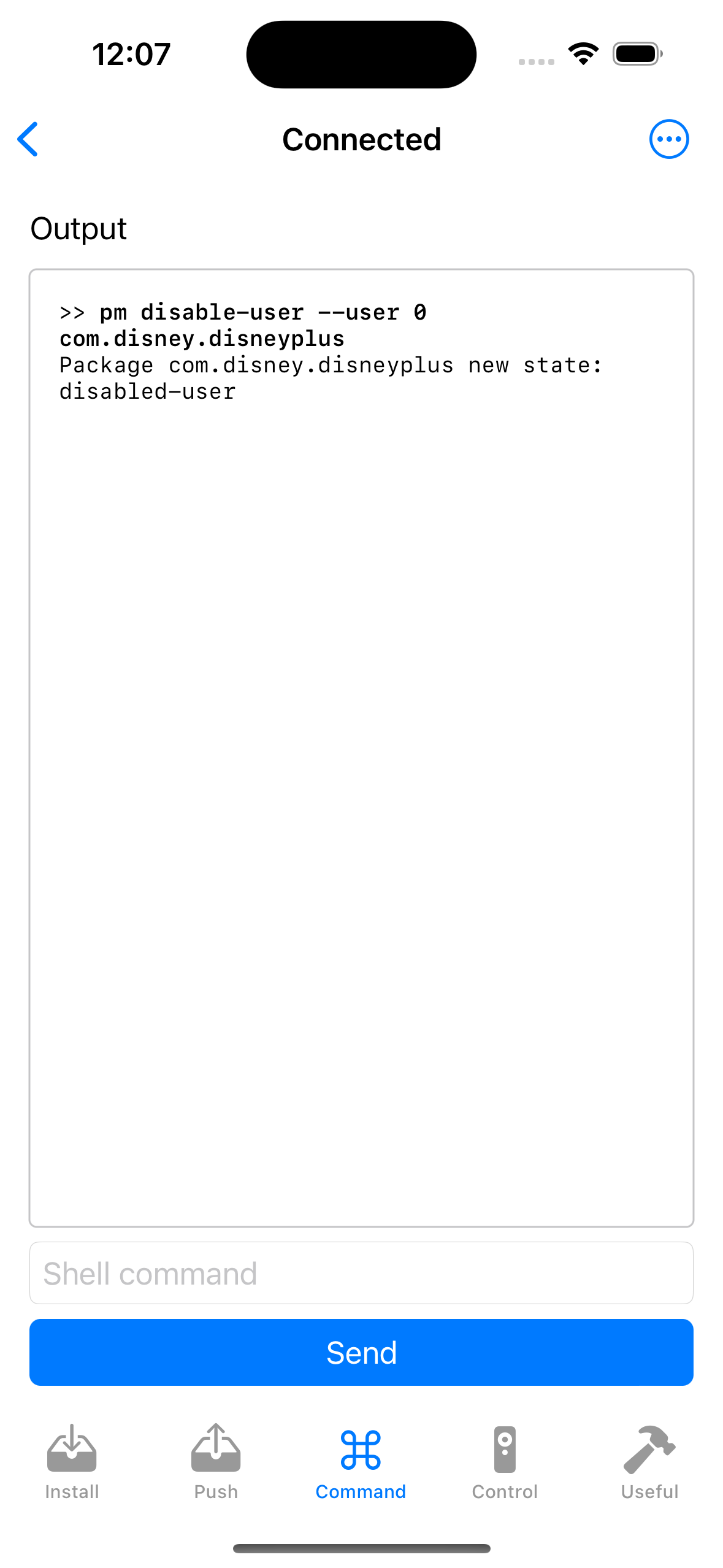A detailed screenshot of a cell phone interface with a white background. At the top left, the time is displayed as 12:07, and the battery indicator shows a full charge. In the middle of the screen, there is a black oval obscuring some content. To the right of this oval are three vertical dots. Below the blacked-out area, there is the word "Connected" with a blue left-facing arrow to its left and a blue circle containing three vertical dots to its right. Further down, the word "Output" is aligned to the left. Under this, there is a light gray-outlined square containing the text "PM Disable User, user" followed by "com.disney.disneyplus." Below this box, the text "package: com.disney.disneyplus" is displayed, followed by "new state…" Underneath is the phrase "disabled user." At the bottom of the page, there is a "Send" button with a blue background and additional clickable options below it.